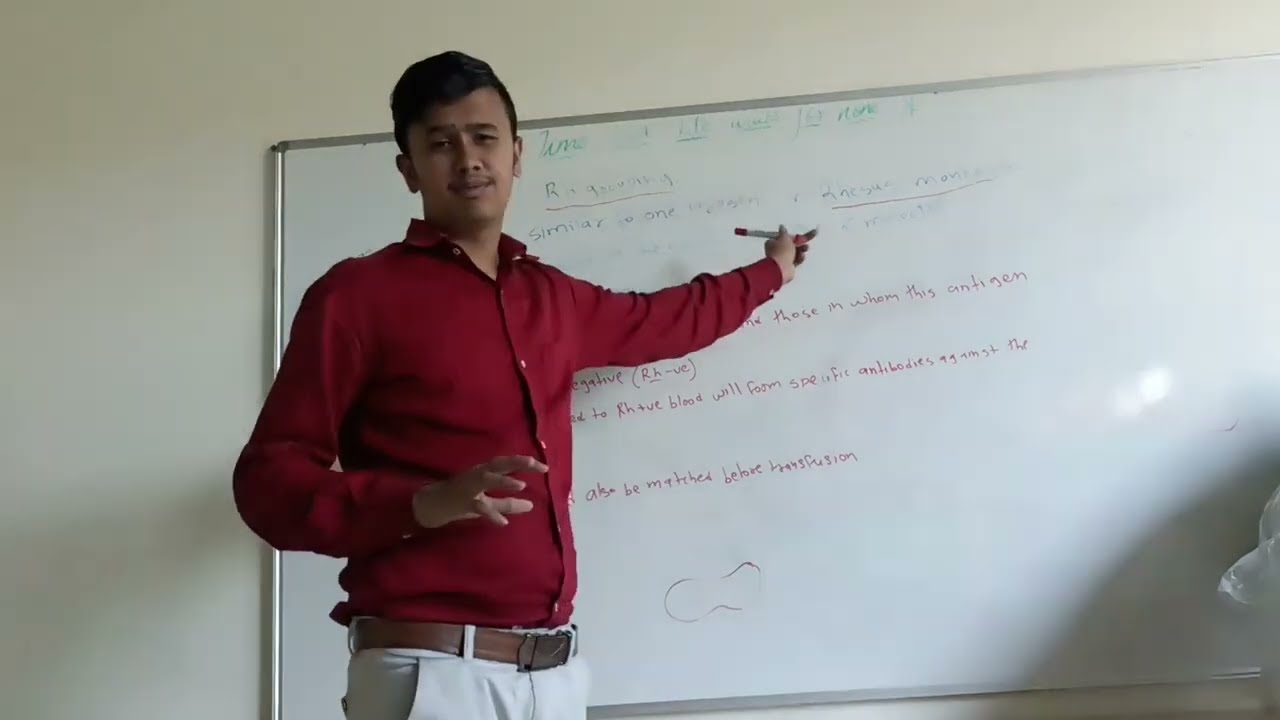This photograph captures an Indian teacher in a classroom setting, seemingly instructing a lesson. The teacher is attired in white pants, a brown leather belt, and a red button-up collared shirt. He is standing next to a large, rectangular whiteboard, which has a silver frame and is mounted on an off-white wall. The whiteboard is covered with green, purple, and red text, which appears to relate to a medical or scientific subject—terms like 'antigen' and 'antibiotics' can be discerned. The teacher, who has short black hair, black eyebrows, and light brown skin, is pointing at the whiteboard with his left hand, holding a red marker. His right hand is bent as if grasping something, and he exudes a confident, almost smug expression as he looks towards the camera. While no students are visible in the image, they may be just outside the camera's view or possibly attending the session online.